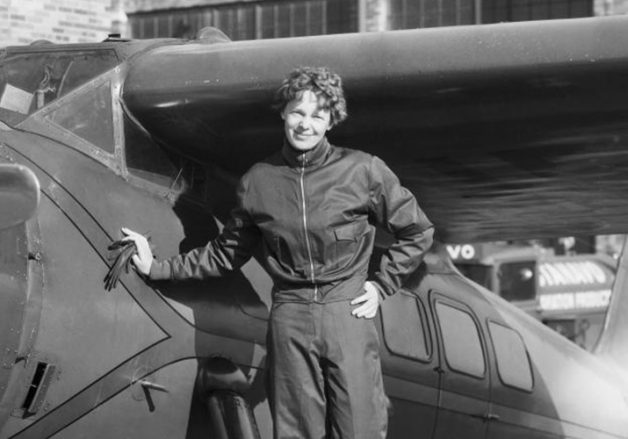This black-and-white photograph captures a historical moment with a woman standing beside an airplane. The image appears aged, likely taking us back to the World War II era or shortly thereafter. The woman, possibly the famous aviator Amelia Earhart, is depicted in a dark windbreaker-style jacket and matching dark pants, attire that provides warmth and suggests a pilot's practicality. With short, cropped curly hair, she is holding a pair of gloves in her hand while resting it against the side of the plane. Her other hand is set confidently on her hip. She stands elevated, as if on a small platform or step, and gazes directly at the camera with a smile. The airplane beside her is relatively large, capable of accommodating multiple people, and she appears to be touching the airplane's window. The photo, horizontal in shape, captures not just a scene but a piece of aviation history.